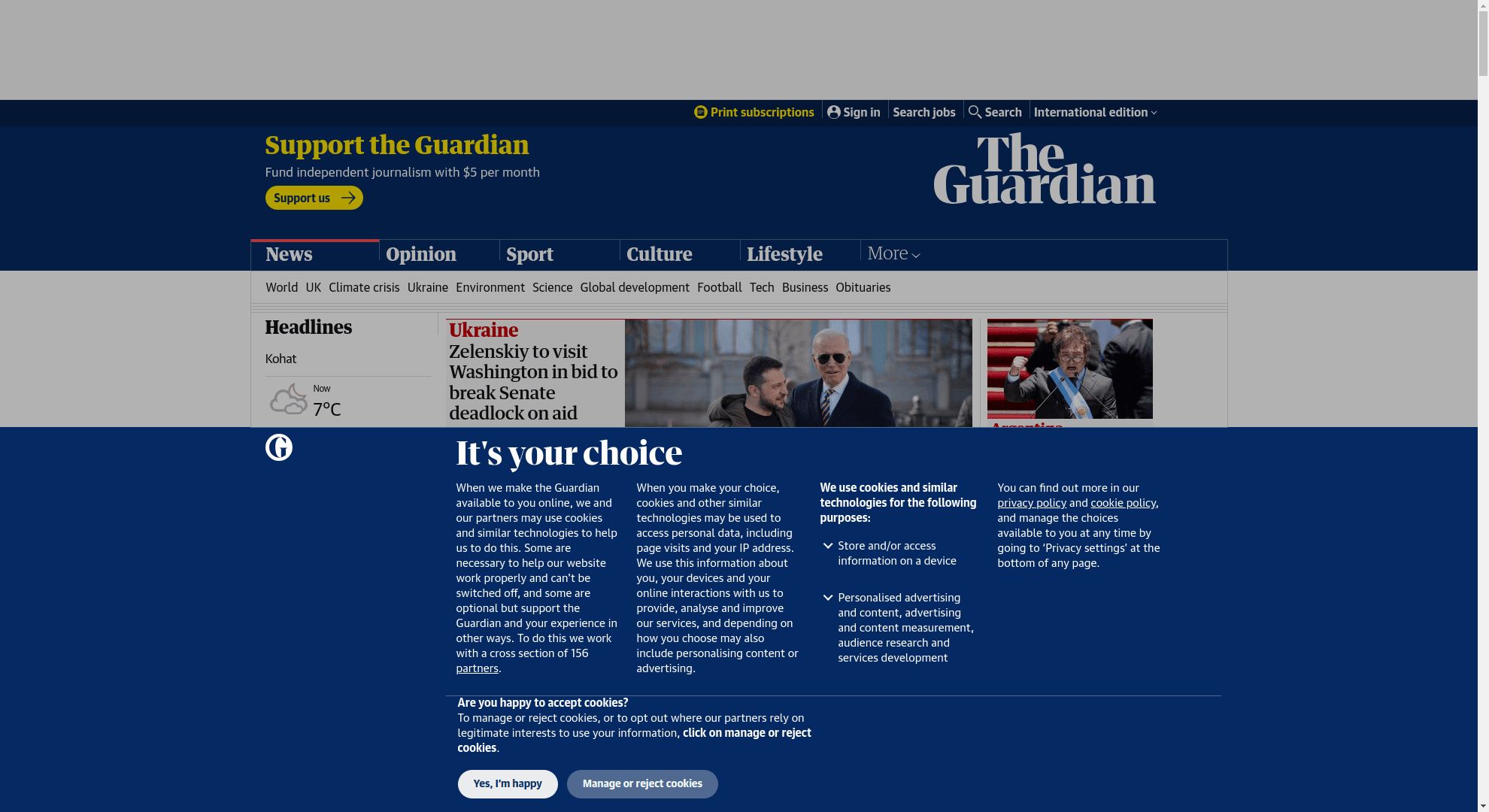This is a detailed screenshot of the homepage of The Guardian website. At the very top, there is a thick gray rectangle spanning the width of the page. Directly below it, there’s a dark blue, almost black, rectangle featuring a yellow section on the left that reads "support the Guardian" in yellow, followed by a line of white text underneath it. Further down, a horizontal yellow oval button stating "support us" in black text with a black right-pointing arrow is prominently displayed.

On the right side of this dark blue header, "The Guardian" is written in large gray letters, with "The" above "Guardian." Beneath this title is a menu bar containing the categories: News, Opinion, Sport, Culture, Lifestyle, and More, with "More" being in light gray and the rest in white.

Below the menu bar, a horizontal gray rectangle contains additional navigational elements. On the left, it says "Headlines," and to the immediate right of this, "Ukraine" is highlighted in red. Under this, a headline reads "Zelensky to visit Washington in bid to break Senate deadlock on aid."

Next to the headline on the right side, there is an image of Ukrainian President Volodymyr Zelensky with U.S. President Joe Biden standing to his right. Adjacent to this is another image featuring a man, though further context isn't provided in the text.

The lower portion of the screenshot shows a dark blue background with bold white large letters in the center stating "It’s your choice." Below this, there are four horizontally aligned paragraphs of smaller white text.